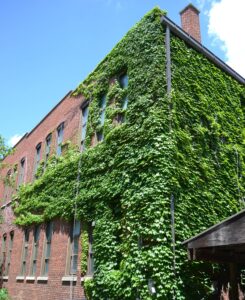In this vibrant, full-color photograph taken outdoors on a mostly sunny day, we see a vertically rectangular image capturing a brick building with a distinct pinkish hue. Viewed obliquely from one corner, the building is mostly covered in lush, green ivy, which even encircles some of the windows. The ivy climbs all the way to the top, where a brick chimney notably extends from the roof. Windows, arranged in groups of three which may be double-hung, are visible on both the top and bottom floors. The pristine blue sky, adorned with white clouds drifting in the upper right corner, adds to the serene atmosphere. Additionally, in the lower right corner, there's a small, gray wooden shed, contributing to the quaint outdoor setting.